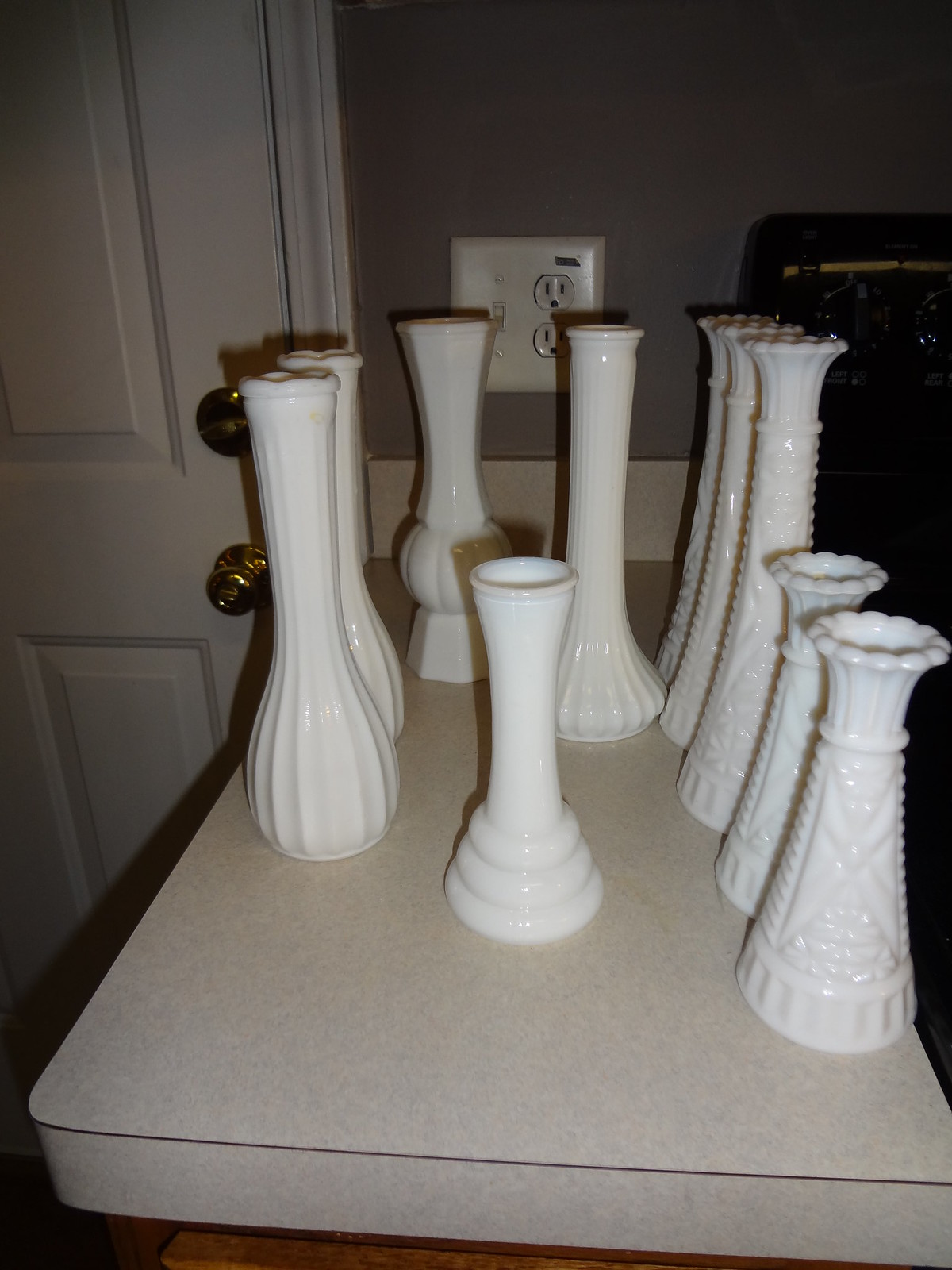This color photograph, taken indoors in a dimly lit room with numerous shadows, features a formica tabletop adorned with a varied collection of white or off-white vases. The table itself, which may be part of a small kitchen countertop, has vases that come in multiple shapes and styles. There are three tall, narrow vases resembling rooks from a chess set and several shorter ones reminiscent of pawns. Additionally, there are vases with varying degrees of curviness and fluted designs, some of which appear to be made of milk glass. Notably, one short vase stands out with three ridges on its base. The background includes a muddily painted putty-colored wall with a light switch and an electrical outlet visible. To the side, there is a closed white door equipped with a gold handle and an upper lock, suggesting it might be an exterior door.